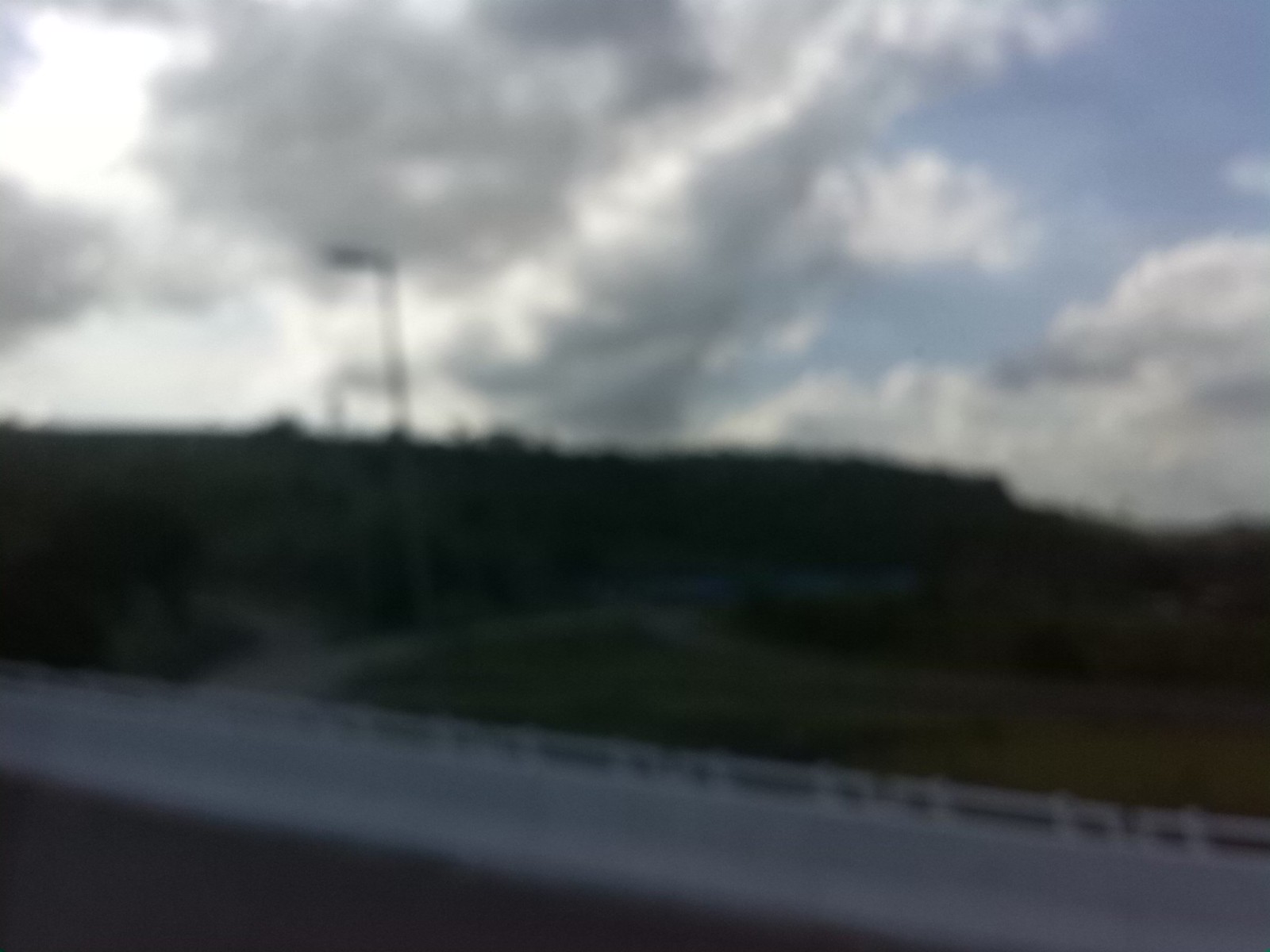This is an extremely blurry landscape photograph that appears to have been taken from a moving vehicle. The image prominently features a large expanse of sky filled with swirling gray storm clouds, partially obscuring the sun. Despite the clouds, there is a glimpse of blue sky in the top right corner. Below the sky, the horizon line meets the land, with a green valley prominently in view and hills in the distance. Stretching horizontally across the lower portion of the image is a gray road, bordered by a small white guardrail or fence. 

A notable feature in the photograph is a metal structure that resembles a streetlight, positioned off-center towards the left. The structure rises vertically before extending horizontally, somewhat square-shaped at the base. The landscape includes patches of green trees, plants, and grass, although these details are difficult to discern due to the poor focus. Additionally, the road in the foreground branches off into what seems to be another road or driveway towards the center-left, creating a complex network.

Overall, the image is cast in a dull light due to the oppressive cloud cover, giving an impression of an overcast or shaded area. Despite the blurriness, the scene vividly captures a dynamic and somewhat somber weather pattern over a sprawling landscape.